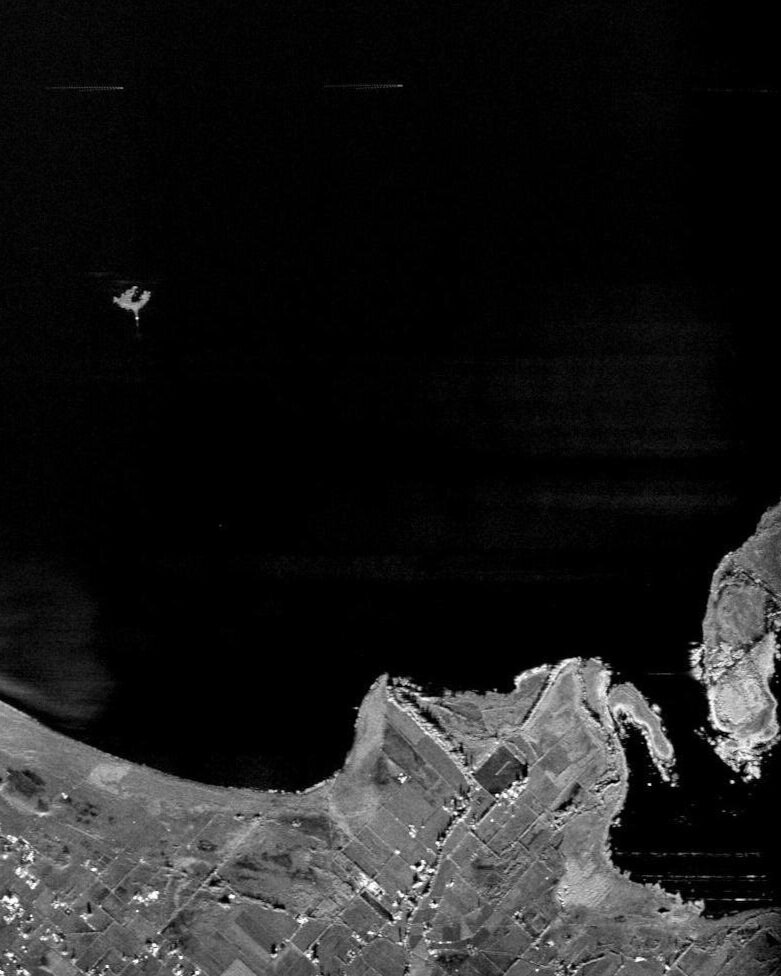The image appears to be an aerial or satellite photograph taken from a very high altitude, possibly from an airplane or satellite. The lower portion of the image showcases a main landmass, clearly segmented into various sections that resemble fields, suggesting a farming community. Dotted within these sections are tiny squares and figures indicative of buildings. Off to the right, a smaller land area extends outward, somewhat finger-like in shape, characterized by dark gray and white hues.

Dominating the upper part of the photograph is a vast expanse of pitch-black, which likely represents water. The stark contrast between the dark water and the lighter land provides a clear delineation of the coastline. Toward the center-right, about halfway up, there's a tiny, isolated island. At the very top of the image, two faint lights with trailing tails are visible, potentially from jets in the sky, adding a dynamic element to the otherwise static scene. Just below these lights, a circular formation with a white bottom and an attached light could be identified as a weather balloon. The entire composition is in black and white, making it difficult to discern finer details such as homes.